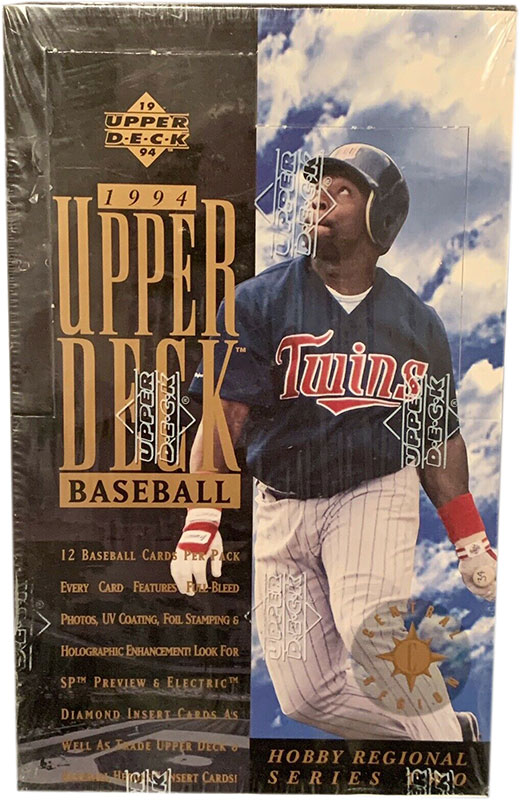The image depicts a vintage 1994 Upper Deck Baseball card pack, still sealed in its original plastic wrap. The pack's design is split into two distinct backgrounds: the left side features a black backdrop with gold lettering that reads "1994 Upper Deck Baseball," followed by "12 baseball cards per pack," and detailed promotion of the card features, including full bleed photos, UV coating, foil stamping, and holographic enhancement. The right side showcases a sky-blue background with white clouds, graced by an African American player from the Minnesota Twins. He is depicted wearing a blue helmet, a navy blue shirt with the word "Twins" in red letters outlined in white, white pants with black pinstripes, and black and white gloves with red accents. The image also lists special card types to look for, such as SP Preview and Electric Diamond inserts, as well as Trade Upper Deck cards. Positioned at the bottom right corner of the pack, it indicates this is part of the "Hobby Regional Series."